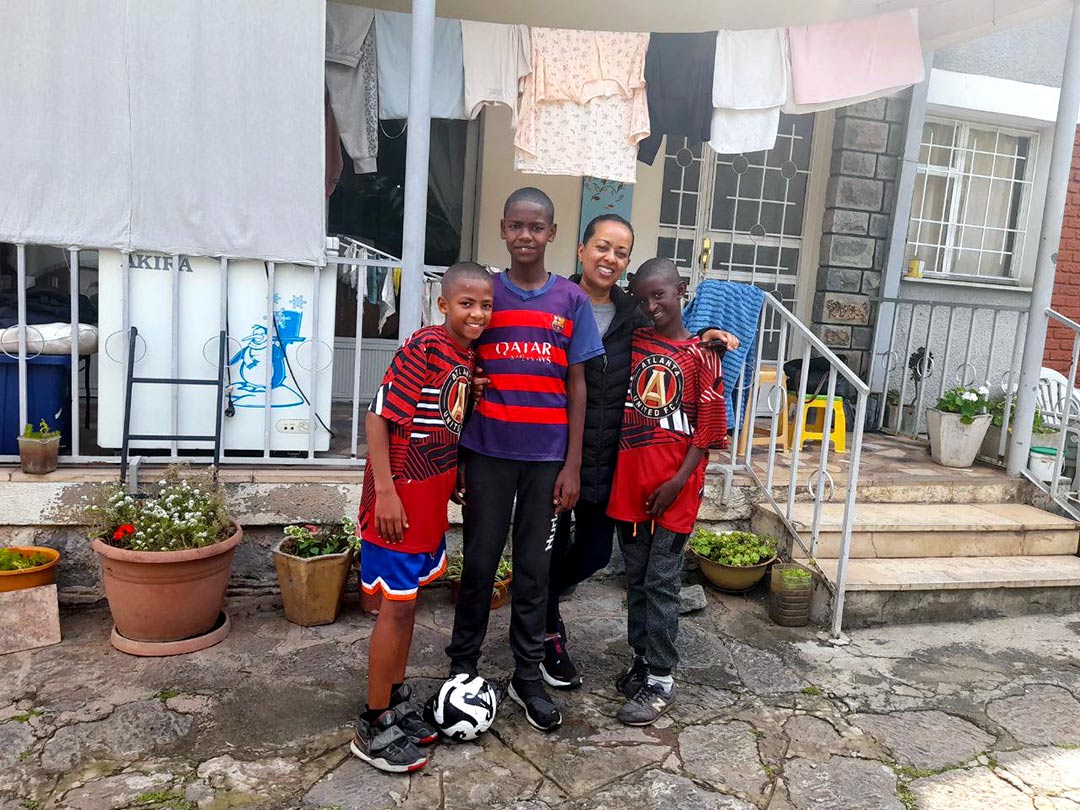This is a horizontal, rectangular photograph of three young boys and an adult woman standing closely together outdoors in front of a grayish-colored house. The boys, who appear to be part of a soccer team, are wearing t-shirts. The young boy on the left is in a red shirt, blue shorts, and black tennis shoes. The taller, darker-skinned boy next to him sports a blue shirt with red stripes and black pants, with a black-and-white soccer ball in front of him. The third boy, who is embraced by the woman, wears a red shirt with a prominent letter "A" on the front and dark pants. The woman, lighter in skin tone and dressed in all black, smiles warmly with her arms around the children. They all stand on a stone patio with steps and a railing adorned with plants, leading up to a porch where clothes are seen hanging to dry.